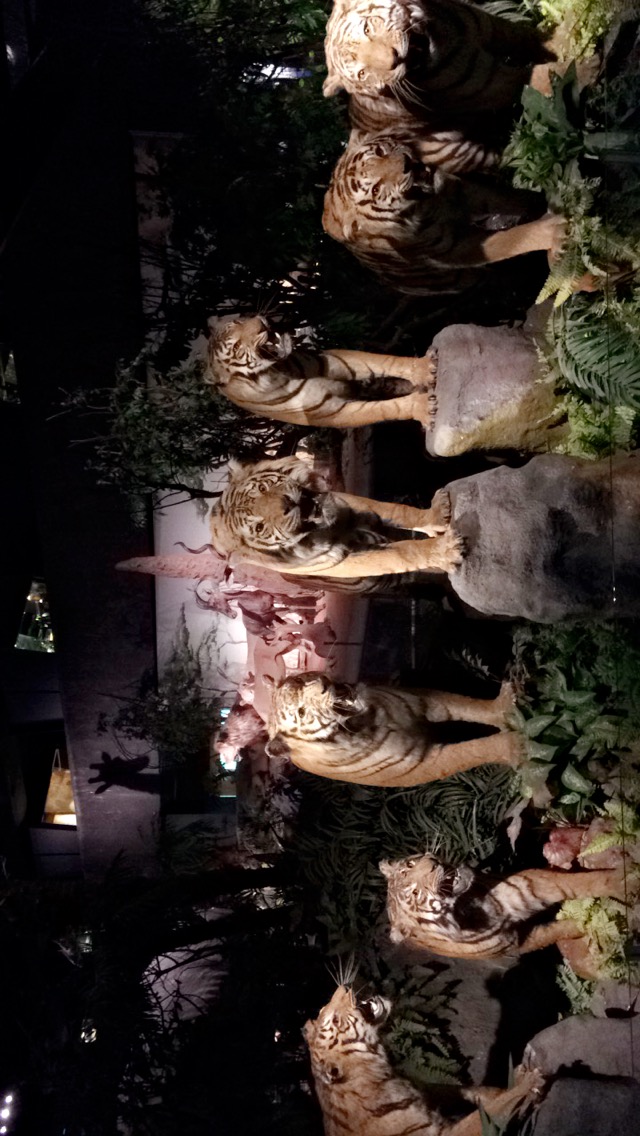The image depicts a museum display showcasing seven lifelike, taxidermied tigers. Each of the vivid orange tigers, marked with black stripes and touches of white on their chests and faces, stands on different heights of faux gray stone pedestals, surrounded by ferns and other lush plant life, evoking a jungle setting. All the tigers are oriented toward the camera with their mouths agape, displaying a slightly fierce demeanor with visible fangs. The scene is illuminated by museum lighting, highlighting the details of the tigers and the textured stones. In the dimly lit background, other exhibits are partially visible, including a silhouetted giraffe, displayed African lions, a gazelle, and artificial trees, creating an immersive but somewhat shadowed ambiance. A doorway and some lights can also be glimpsed amid the darkened environment.